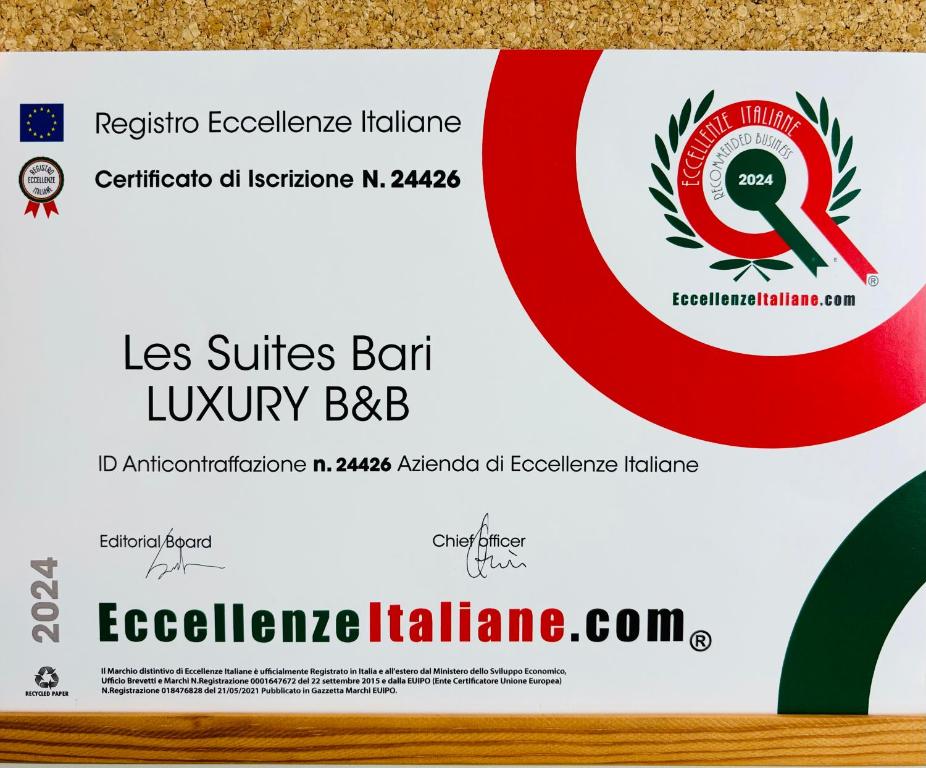This image features a close-up of a business card, seemingly placed on a corkboard with a modeled light brown and tan header and a light brown wood grain border at the bottom. In the top left corner of the business card, there's a blue square with a logo containing red dots and a circular emblem with two red ribbons nearby. Near this emblem, the card reads "Registro Excellenze Italiane Certificato di Iscrizione North 24426." In the central area, prominently displayed in black text, it states "Les Suites Bari Luxury B&B." Below this, smaller text includes "ID Anticontroversione 24426" and "Asciende di Ecolinse Italiante." Towards the bottom, a website address in Italian, "ExcellenzeItalien.com," is printed in red and green. The upper right-hand corner of the card features a conspicuous, thick half-circle with a red outer ring, a white middle ring, and a green center surrounded by laurel leaves. In the lower right-hand corner, a quarter arc of a dark green circle is visible. Additionally, the bottom left corner of the card has gray text indicating the year "2024." The card also includes signatures labeled as from the Editorial Board and Chief Officer, written in black pen.